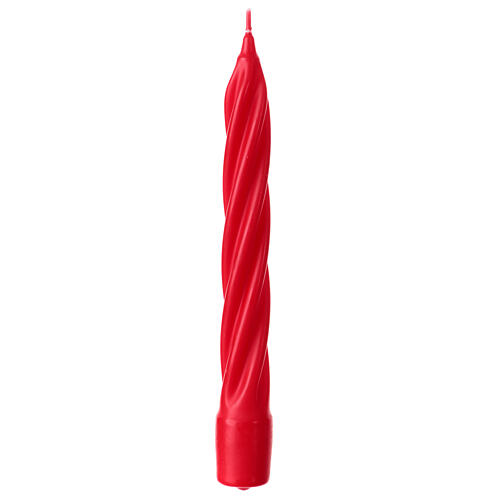This image features a long, skinny, cylindrical, red candle known as a taper candle, specifically designed with a spiral twist that gives it an elegant and visually pleasing shape. The twist spirals clockwise from the pointed top down to the smooth base, where it would fit securely into a candle holder. The candle has not been burned, as indicated by the wax-covered wick at the tip. The entire candle, including the wick, is a lighter red hue. It stands upright on a pristine white background, centered in the frame. The professional lighting highlights its distinctive twisted design and smooth base, making it suitable for both decorative and celebratory purposes, such as being used on a birthday cake.